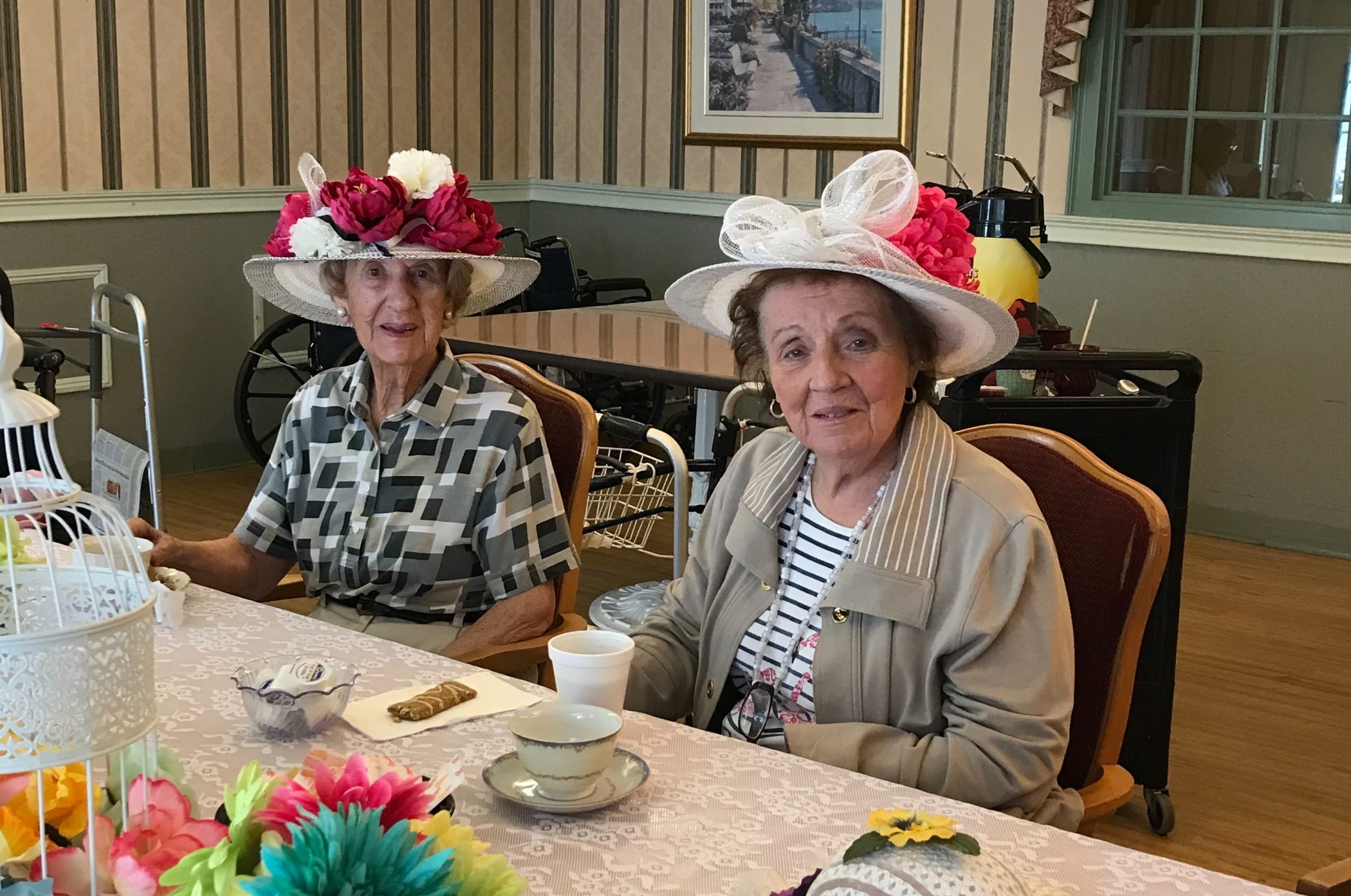In a cozy dining area, likely in a nursing home, two elderly women sit at a long table enjoying a cheerful tea time. Both women, estimated to be in their 70s or 80s, are donned in wide-brimmed white hats adorned with an array of vibrant silk flowers in colors such as red, dark pink, and white. The lady on the right also sports a fluffy white bow on her hat, paired with a gray jacket featuring some stripes, while the lady on the left wears a geometric print shirt. They sit in wooden chairs with maroon backs, facing a table covered with a pink floral tablecloth. 

In front of them are ceramic teacups, a plastic coffee cup, individual creamers in a glass bowl, and a granola bar. Behind them, a black commercial beverage cart showcases two yellow carafes. The table’s centerpiece is a decorative birdcage surrounded by colorful flowers, adding to the room’s inviting atmosphere. The surrounding area features a lower gray wall and an upper wall with peach and gray stripes, adorned with a painting. Nearby, a walker and a wheelchair are parked side by side, in view. The women, gazing contentedly at the camera with amused expressions, are participating in what appears to be a special luncheon in this warm and thoughtfully adorned space.